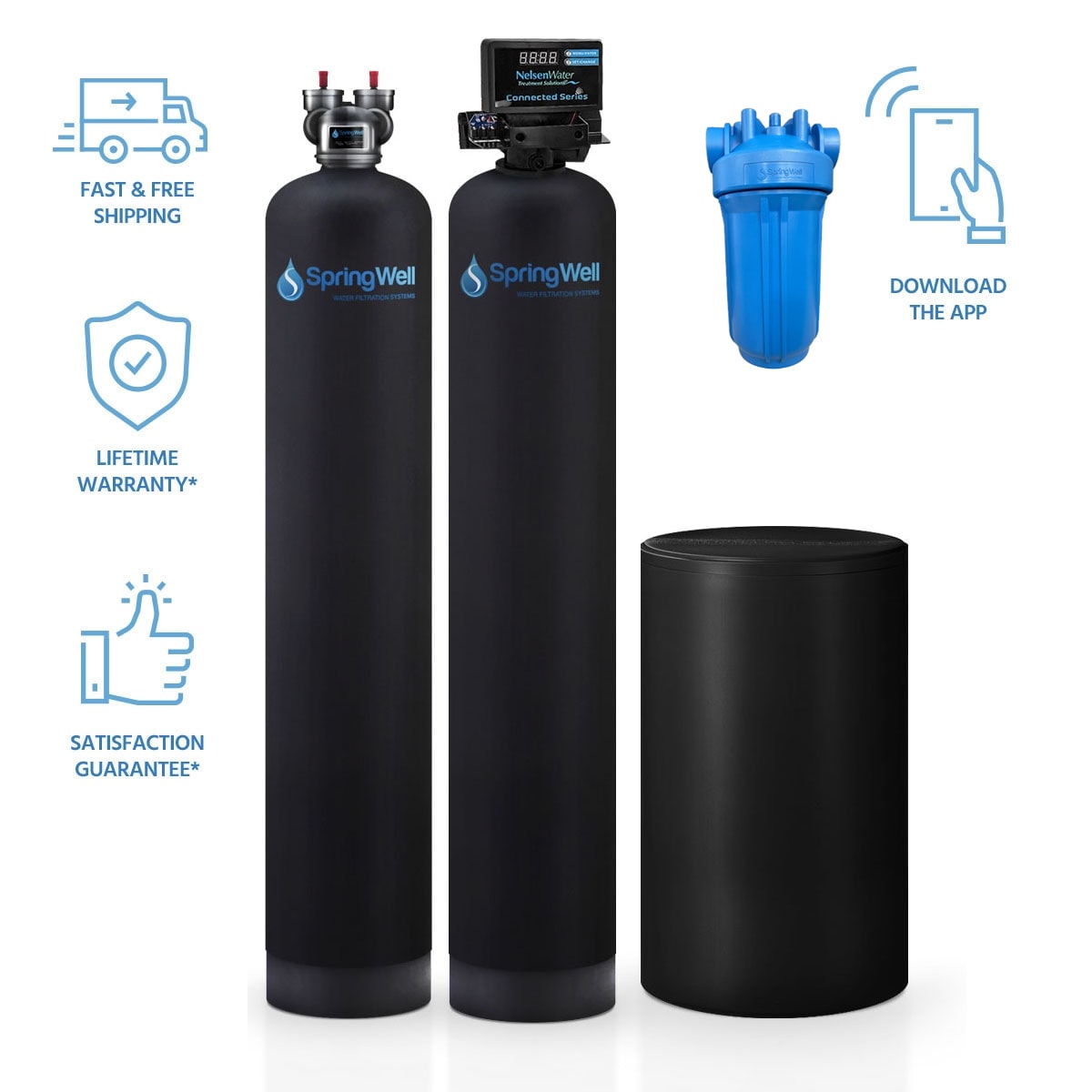This image appears to be an advertisement for Springwell water filtration systems. Dominating the scene are two large, black water tanks adorned with the white Springwell logo, which includes a water drop icon featuring an 'S'. The first tank stands without any additional attachments, while the second tank is topped with a small control box.

To the right of these tanks, a smaller, sky-blue container and a round canister with a flat top can be seen. The left side of the image features a truck icon accompanied by the text "Fast and Free Shipping" in light blue. Below this, a shield icon with a checkmark prominently displays "Lifetime Warranty," followed by a thumbs-up icon with the promise "Satisfaction Guaranteed."

In the top right corner of the image, a hand icon holding a phone with several lines emanating from it signifies connectivity, and directly below this, the text encourages viewers to "Download the App." The background is clean and minimalist, focusing attention on the Springwell products and their associated benefits.